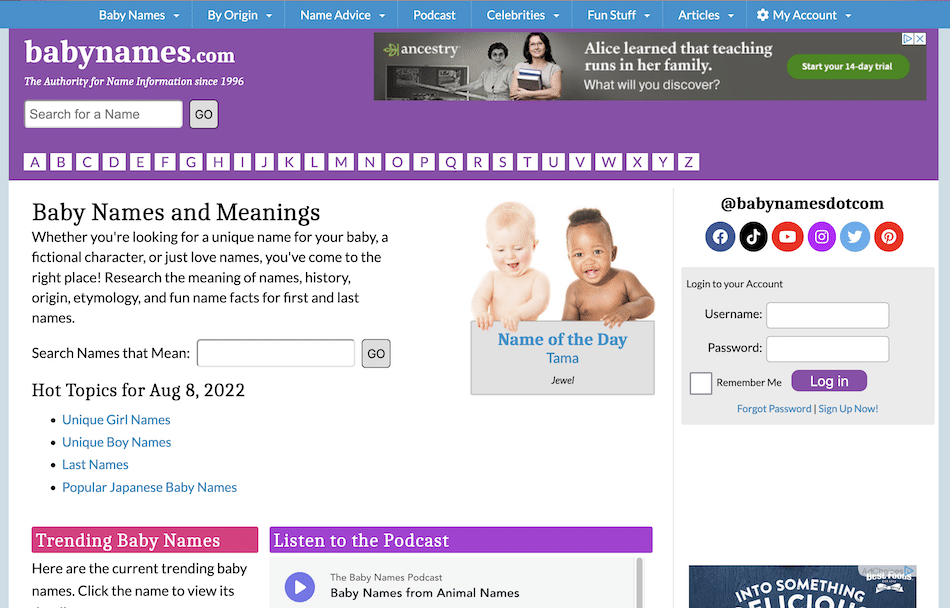The image features a screenshot of the website BabyNames.com, a respected authority on name information established in 1996. Prominently displayed at the top is an advertisement for Ancestry.com, which highlights a user's discovery of teaching running in their family roots.

Central to the image is a distinctive purple box that hosts the search function for names, accompanied by the alphabet from A to Z. Just below this in a white box, the website’s main features are detailed: information about baby names and their meanings. The text explains that whether someone is searching for a unique name for their baby, a fictional character, or simply loves names, BabyNames.com is the ideal resource. Users are invited to research the meaning, history, origin, and fun facts about first and last names and to utilize a versatile search tool that accommodates both name-to-meaning and meaning-to-name queries.

Highlighted on the site are the "Hot Topics" for August 8th, 2022, listed as unique girl names, unique boy names, last names, popular Japanese baby names, and trending baby names. The trending names section instructs users to click on the names to explore further details, although the information appears to be cut off in the screenshot.

Featured as the "Name of the Day" is Tama, spelled T-A-M-A, meaning "Jewel," showcased by an image of two babies holding up a sign with the name. Lastly, the website's login area indicates that users need an account to access personalized features, prompting them to enter a username, password, and an option to remember login details for future visits.